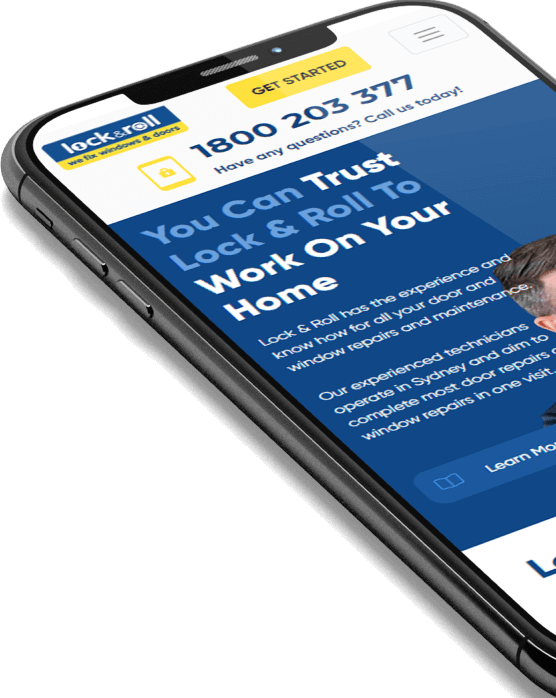The image features a black smartphone laid diagonally across the frame, displaying a website interface related to window repair services. At the top left corner of the screen, the text "Lock and Roll, Fix Windows and Doors" is prominently featured, with the phrase "Lock and Roll" set against a blue background with white text, while the accompanying tagline rests on a yellow background with blue text. To the right of this section, there is a yellow "Get Started" button and a white "Menu" button. Directly beneath these elements, a contact phone number, 1-800-203-377, is displayed in blue text with the message, "If you have any questions call us today." Following this, a blue section assures customers that they can trust "Lock and Roll" to work on their home, with "You can trust Lock and Roll to" in light blue text and the rest in white. Below this reassurance, there is a passage of text in white, set against a solid white background. The overall composition of the image ensures clarity and emphasis on the key website elements designed to instill customer confidence and facilitate easy navigation.